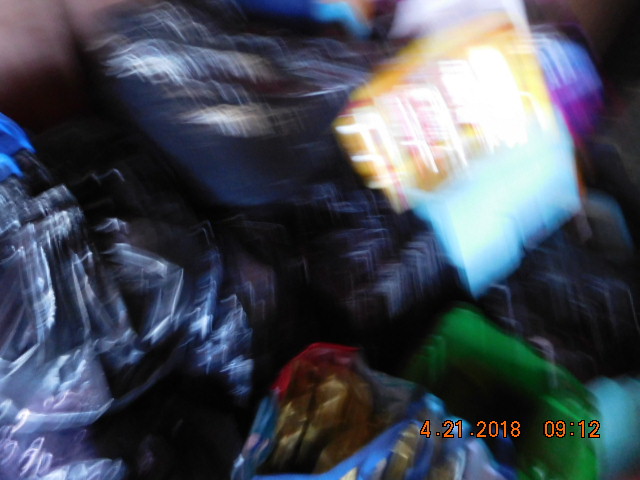A highly indistinct and blurry photograph capturing what appears to be a jumble of various images, making it challenging to identify any specific objects or subjects. The photograph features a prominent time and date stamp at the top reading "4/21/2018 at 9:12." In the central portion of the image, there is a dark area that might represent a person wearing a black jacket, with noticeable white reflections akin to those of a trash bag. The bottom of the image displays a mixture of blues, yellows, and reds, resembling pieces of fabric. Additionally, a green object is visible towards the bottom right corner. In the upper right-hand corner, there is a small gray dot, though its significance or exact nature remains unclear.